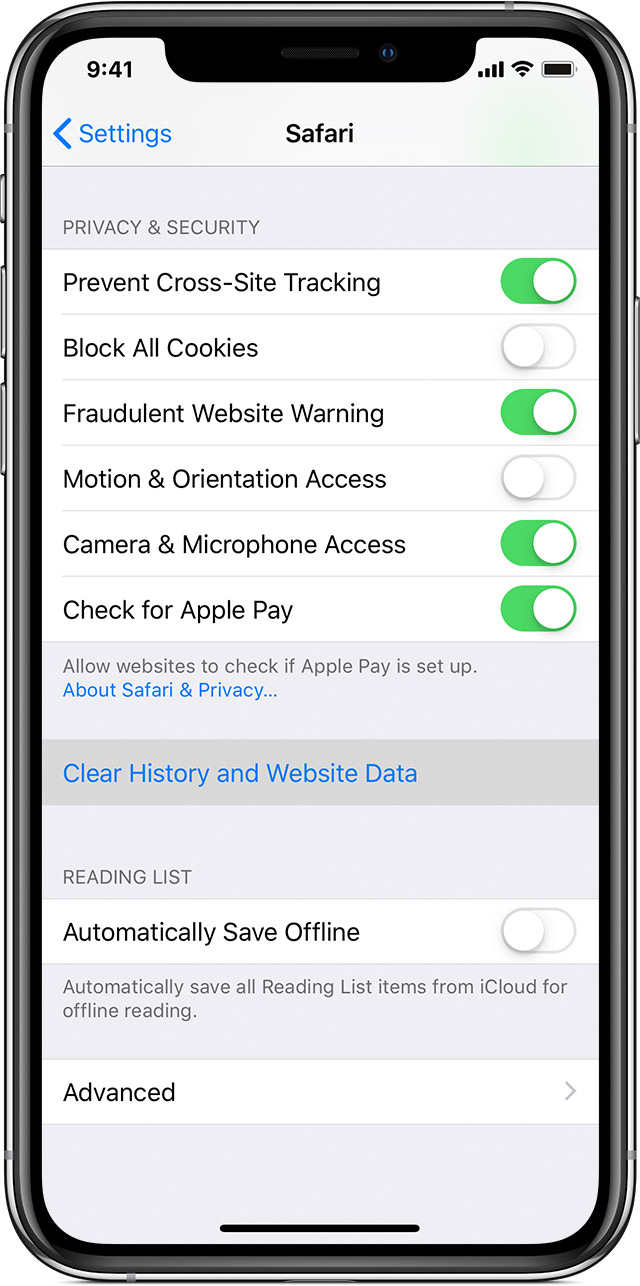The photograph captures the screen of a black iPhone, framed distinctly by its body and edges, with visible buttons on both the left and right sides. The screen displays the "Settings" menu, specifically the "Safari" settings section.

At the top left, a blue text labeled "Settings" is accompanied by a left-pointing arrow. Centered at the top, "Safari" is written in small black letters. Just below, in small gray letters, is "Privacy and Security," followed by a list of options with corresponding toggle switches.

The first option, "Prevent Cross-Site Tracking," shows a green toggle switch indicating it is turned on. The second option, "Block All Cookies," has a white toggle switch, signaling it is turned off. The third option, "Fraudulent Website Warning," has its toggle switch set to on. "Motion and Orientation Access" follows with its toggle switch off. The "Camera and Microphone Access" option is toggled on, as indicated by the green switch. Lastly, the "Check for Apple Pay" option also shows a toggle switch in the on position.